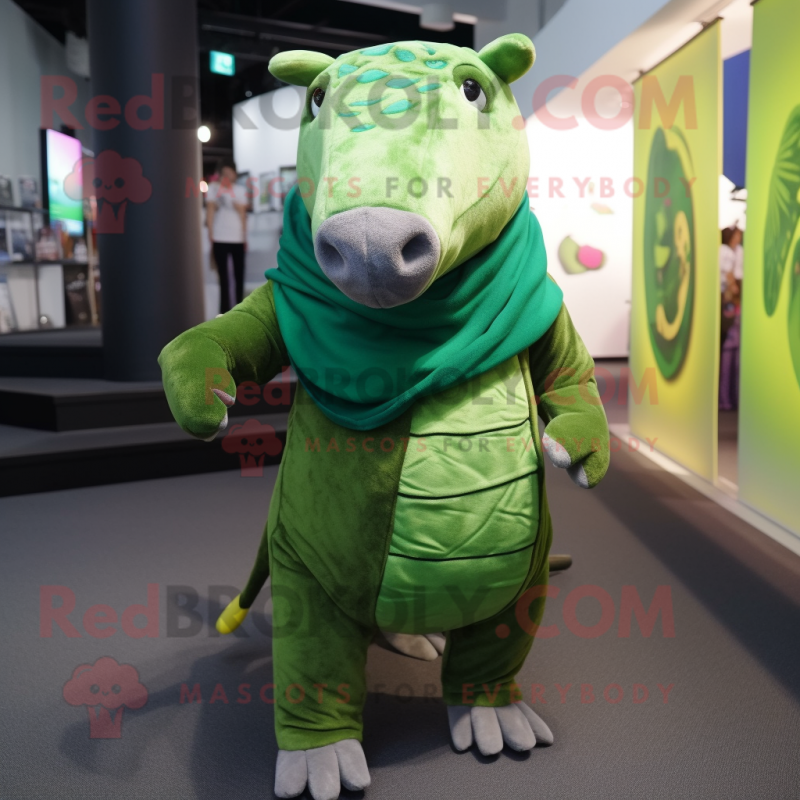The photo, taken indoors, captures a character in a vibrant green mascot costume, potentially a hybrid between a pig and a dinosaur based on its various features. The costume's details include a green body with a matching large scarf, a gray snout suggestive of a pig, and small green ears. The feet are white with distinctive purple toes, while the tail is green with a small yellow knob at the tip. Surrounding the mascot, the setting includes brownish carpet flooring, a staircase, a round pillar, and a person standing blurred in the background. There are green-tinted posters and screens with the text "redbroccoli.com mascots for everybody" or "for every occasion" visible as a watermark across the image.